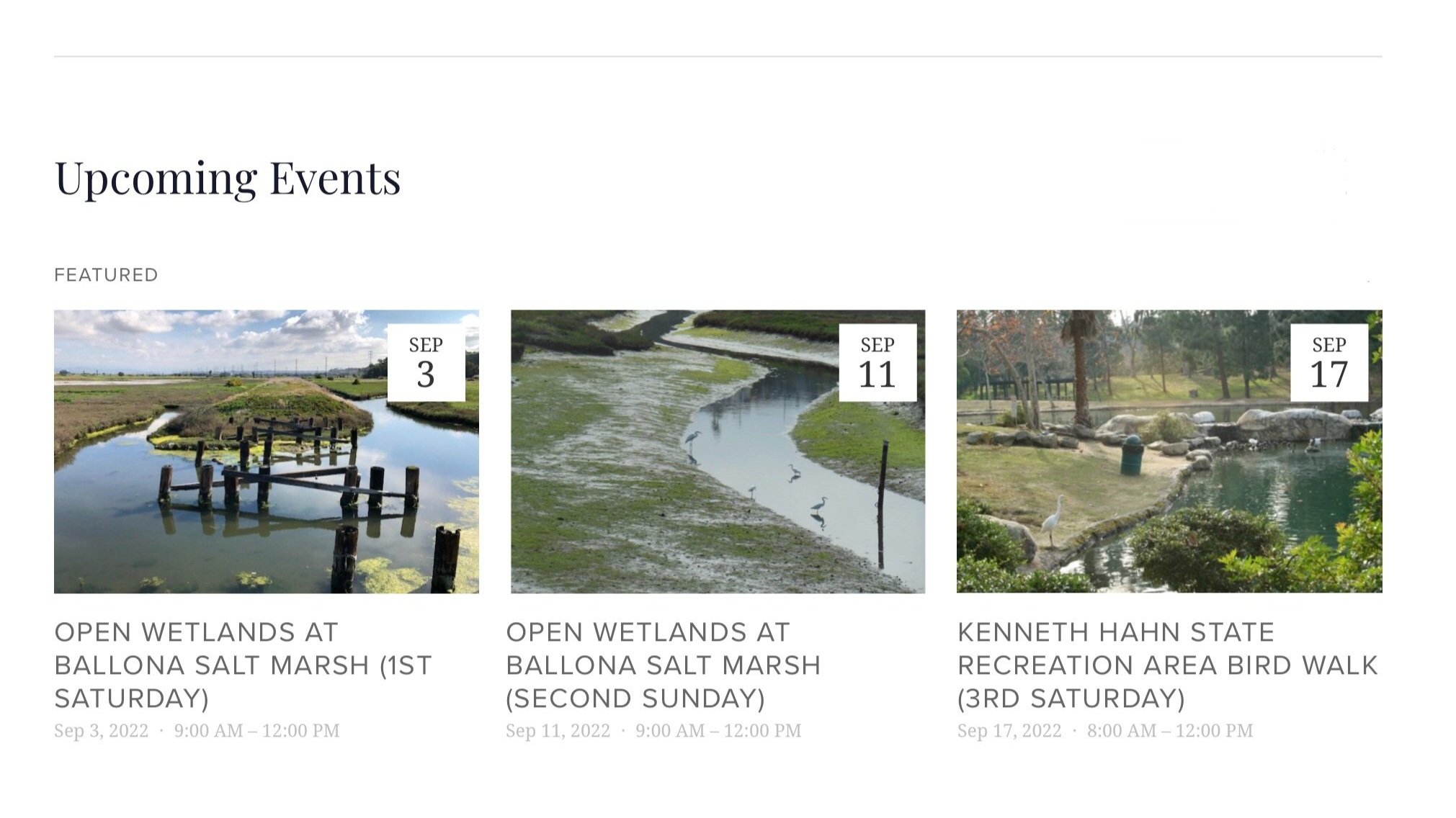This screenshot captures a section from a website under the heading "Upcoming Events" located in the top left corner in black text. Below this heading, the text "Featured" is displayed in gray. The section showcases three event listings, each represented by an image with pertinent details.

1. **Event 1: Open Wetlands at Bologna Salt Marsh**
   - **Image Description**: A daytime scene of wetlands featuring a somewhat swampy area with wooden poles emerging from the water.
   - **Event Date**: September 3, indicated in a small white box in the upper right corner of the image.
   - **Event Details**: "Open Wetlands at Bologna Salt Marsh - First Saturday, September 3rd, 2022, 9 a.m. to 12 p.m."

2. **Event 2: Open Wetlands at Bologna Salt Marsh**
   - **Image Description**: Another perspective of a swampy marshland area.
   - **Event Date**: September 11, indicated in a small white box in the upper right corner of the image.
   - **Event Details**: "Open Wetlands at Bologna Salt Marsh - Second Sunday, September 11th, 2022, 9 a.m. to 12 p.m."

3. **Event 3: Kenneth Hahn State Recreational Area Birdwalk**
   - **Image Description**: A serene park setting with a creek meandering through green fields and a lush green forest.
   - **Event Date**: September 17, indicated in a small white box in the upper right corner of the image.
   - **Event Details**: "Kenneth Hahn State Recreational Area Birdwalk - Third Saturday, September 17th, 2022, 8 a.m. to 12 p.m."

Each event listing features gray text beneath the corresponding images, providing descriptions and specific details about the location, date, and time of the upcoming events.